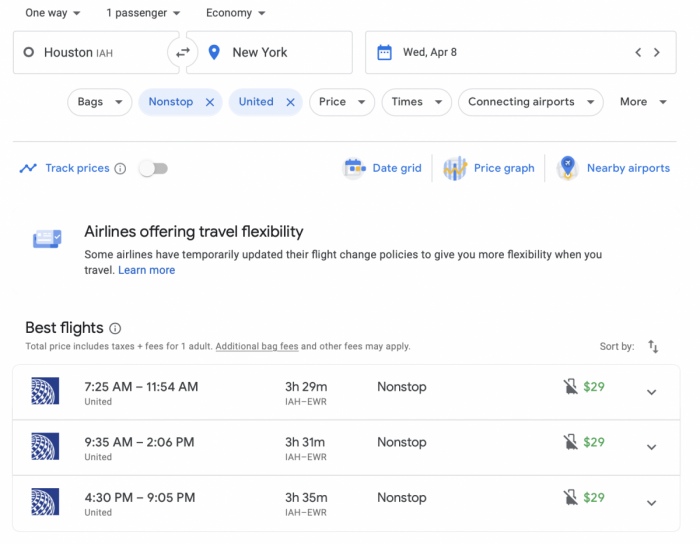**Caption:**

A United Airlines economy flight from Houston to New York is scheduled for Wednesday, April 8th. This non-stop flight is part of a broader trend where airlines, including United, offer a range of flight options with flexible travel policies to accommodate passengers’ needs during these uncertain times.

Travelers have various options to manage their schedules and preferences. United Airlines promotes competitive pricing, with a highlighted route priced at $29 for non-stop flights. For example, a flight departs at 9:35 AM from IAH (George Bush Intercontinental Airport) and arrives at 2:06 PM at EWR (Newark Liberty International Airport), totaling a duration of 3 hours and 31 minutes. Another option is a flight that leaves at 4:30 PM, landing at 9:05 PM, taking 3 hours and 35 minutes.

Please note that the total price includes taxes and subsidies but additional baggage fees might apply. The background theme of the flight offerings emphasizes a subtle, light ambiance, promoting a calm and hassle-free travel experience.